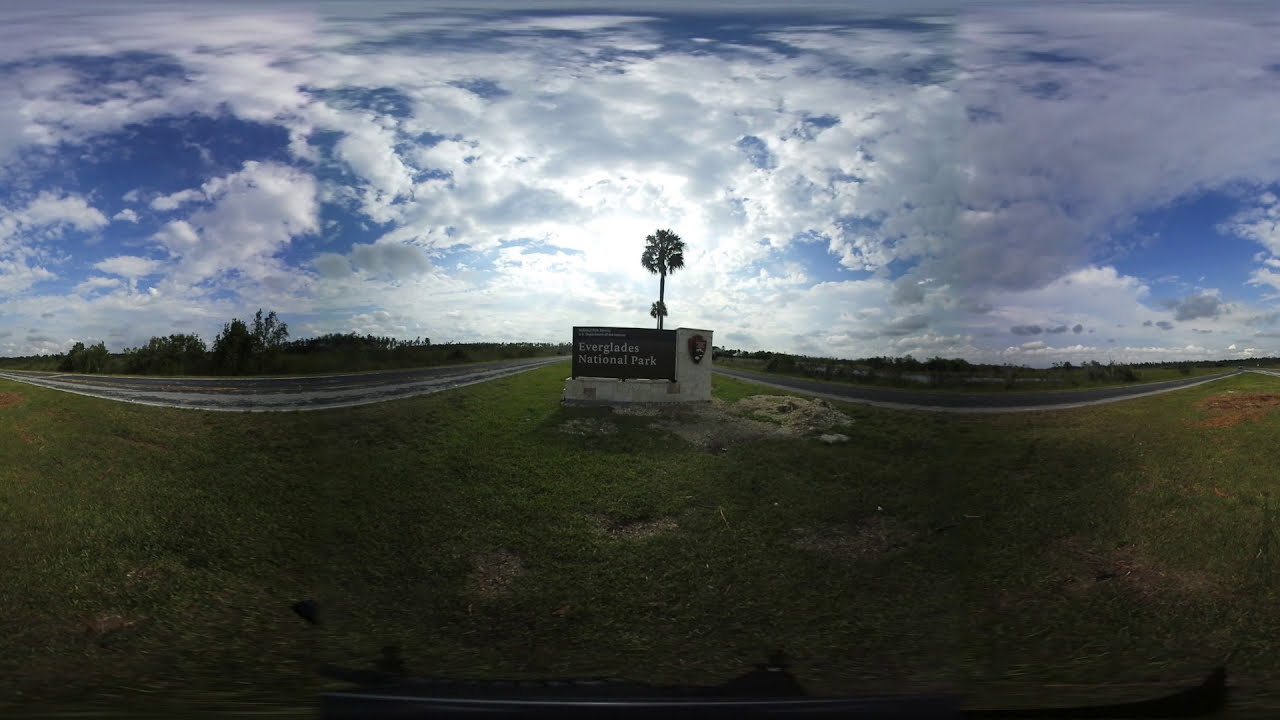The panoramic photo showcases a sign for Everglades National Park prominently in the center. The sign itself is brown with the text "Everglades National Park," mounted on a distinct white stone foundation and accompanied by the National Parks logo on the right side. The composition of the sign is enhanced by tall palm trees directly behind it, adding to the tropical atmosphere of the scene. Surrounding the sign is a mixture of flat grassy areas, some patches lush and green while others are sparse with signs of dead grass. In the background, the landscape transitions into a roadway visible on both sides of the image, with additional trees more concentrated to the left side. The upper half of the image is dominated by a vibrant blue sky teeming with various types of clouds — from puffy white clusters to darker, closer formations. The photo benefits from dramatic lighting, with the sun partially obscured by clouds, creating a slightly backlit effect on the sign and casting a bright highlight behind the palm tree.